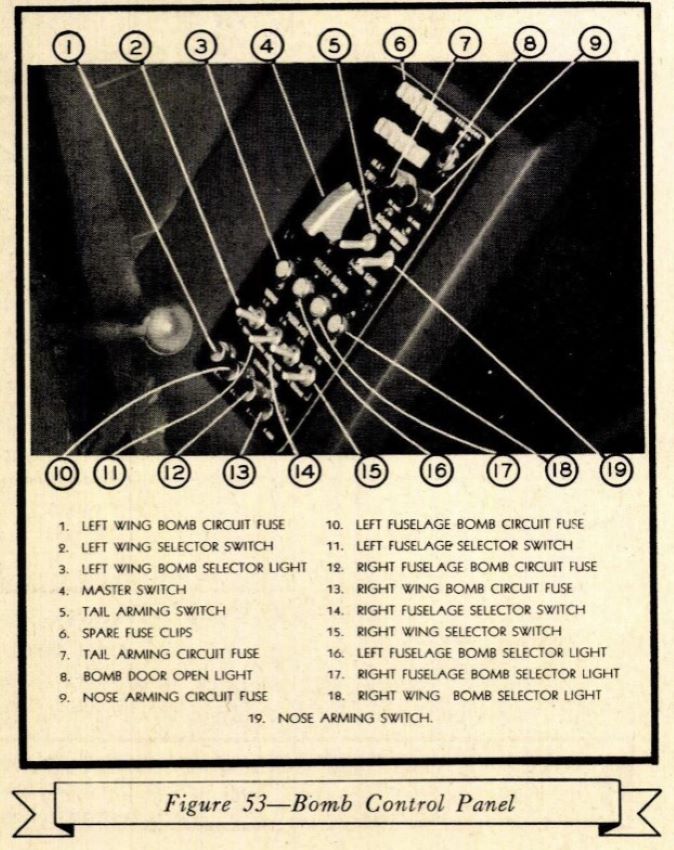The image is a scanned black-and-white photograph from a yellowed page, likely originating from a magazine or instructional pamphlet dating back several decades. It depicts Figure 53: Bomb Control Panel, a detailed vintage diagram. The photograph shows a bomb control panel featuring numerous switches, buttons, and lights, each labeled with a number from 1 to 19. These numbers are connected to parts of the control panel through drawn lines. Below the image, there is a corresponding list explaining each numbered part, such as 1. Left Wing Bomb Circuit Fuse, 2. Left Wing Selector Switch, and 19. Nose Arming Switch. The panel is elaborately designed to include various critical components necessary for bomb control operations, providing a comprehensive visual and textual guide to this complex instrument.